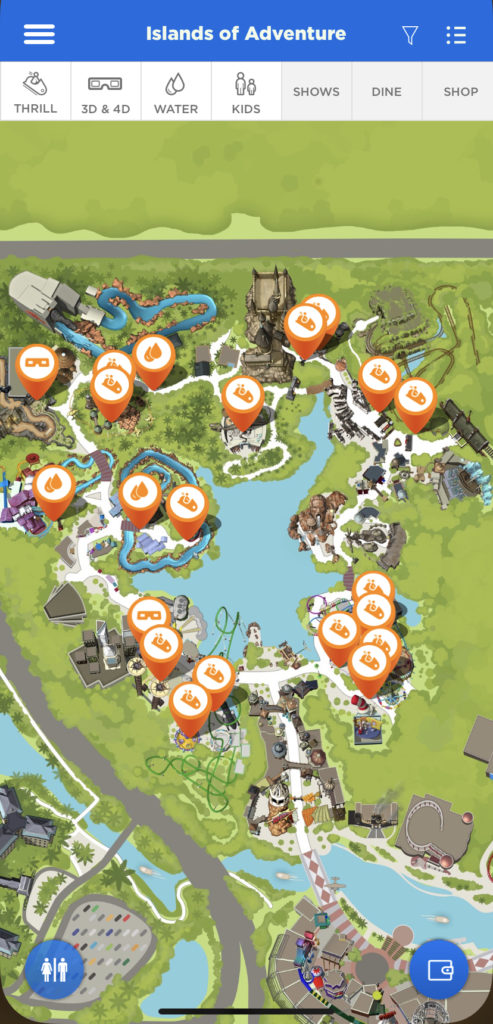The image features a vast expanse of grass dominating the foreground. On the left side, a serene blue river meanders through the landscape. Adjacent to the river stands a gray building, possibly an office or residential structure. Scattered around are icons in shades of orange, likely indicating different functionalities or points of interest on the digital display overlaying the image. 

Further to the right, urban elements such as streets and parking lots filled with cars are visible, showcasing the transition from natural to built environments. The top left corner captures another segment of the river, seamlessly integrating nature with the metropolitan area. The overall scene is part of an interactive digital map interface, featuring various sections and interactive elements, possibly related to navigation or location-based information. At the bottom right, an icon that resembles a wallet hints at financial or transactional capabilities within the map interface.